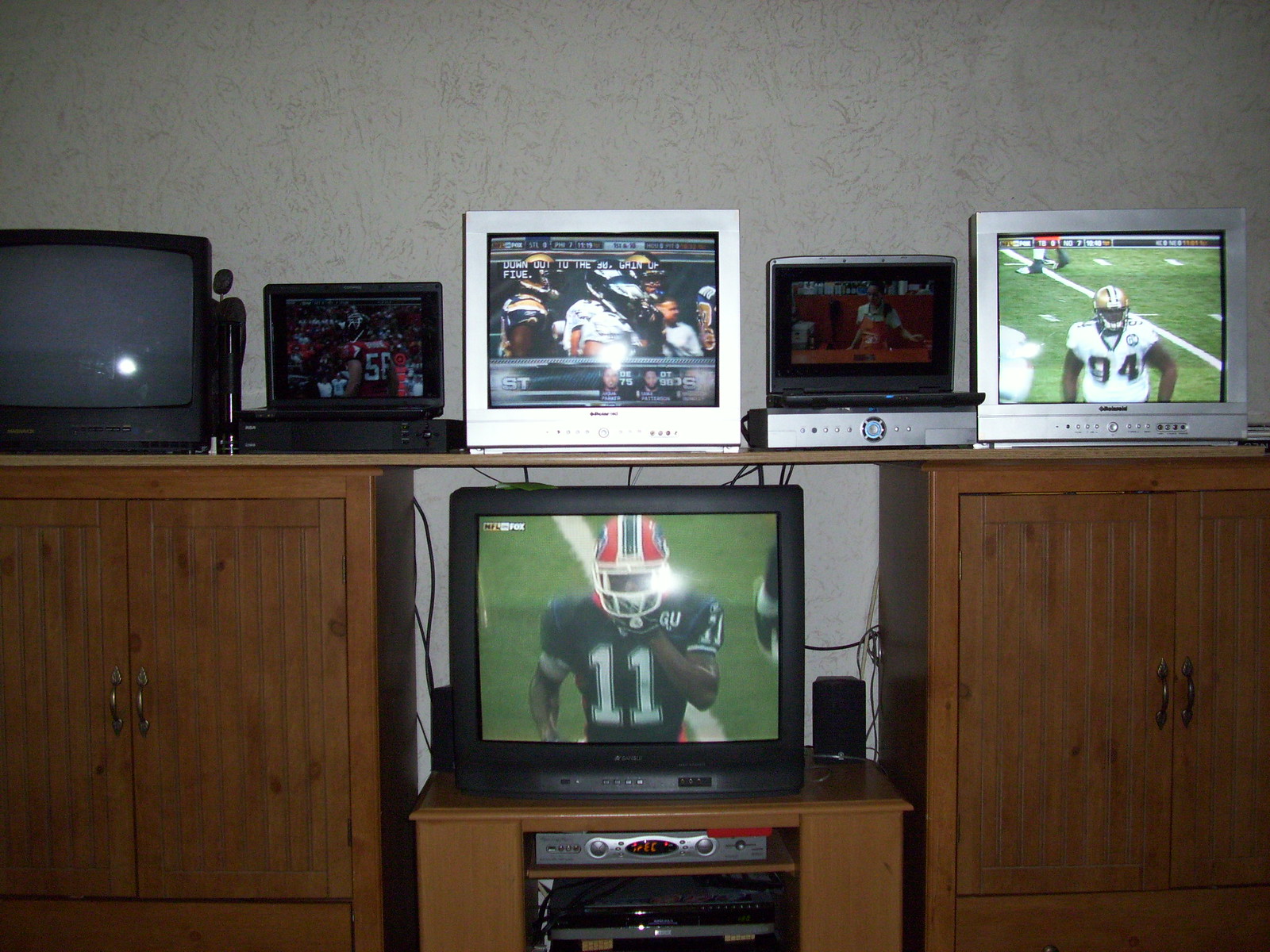The image depicts an old-school sports entertainment center within a home. At the bottom of the picture, two brown wooden cabinets with French door-style handles flank a central wooden stand. This stand supports a large, old-fashioned CRT TV displaying a football game with player number 11 prominently in the frame. Beneath this TV, on the stand, sits either a DVD player or a VCR. Above the cabinets, a wooden board holds a total of five additional screens. Starting from the right, there is a smaller CRT TV broadcasting a football game, similar in style to the main TV, with the player close to the camera. Next to it is a portable TV that appears to fold down into its case, likely a DVD player. Another CRT TV follows, showing a different sporting event, and beside it, another portable TV of similar design. The leftmost CRT TV, encased in black, is turned off. All operational TVs are tuned into various football games, illustrating a setup designed for watching multiple sporting events simultaneously in a vintage style.